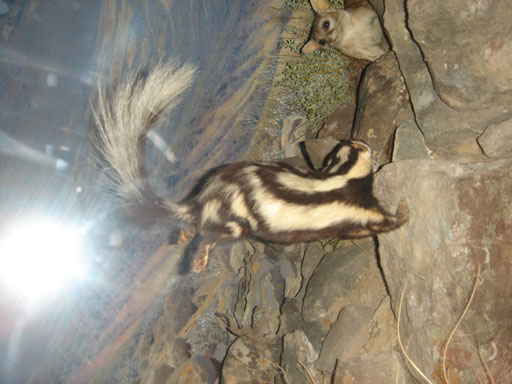The photograph captures a dramatic scene featuring a skunk in mid-jump, seen in profile, with distinct black and white stripes that are more detailed than usual. The skunk's long, bushy tail is prominent, with white underneath and black on top. It appears to be performing a dynamic handstand on a reddish-tan rock, as it braces for impact with its front paws. Surrounding the skunk, a variety of rocks are scattered, adding depth to the scene.

In the top center of the image, a fox-like marsupial with pointy ears and black eyes observes the skunk, sitting on one of the rocks. The animal's coat is brown, contrasting with the skunk's vivid markings.

This image, likely taken indoors as part of a museum display due to the flash reflection and staged appearance, includes a bright circular light source at the bottom left, which partially obscures the background. The backdrop, possibly a photographic representation, shows an open field with distant bushes and trees, adding to the naturalistic setting of the display. The photograph might be rotated 90 degrees, creating the illusion of different orientations of movement for the skunk.